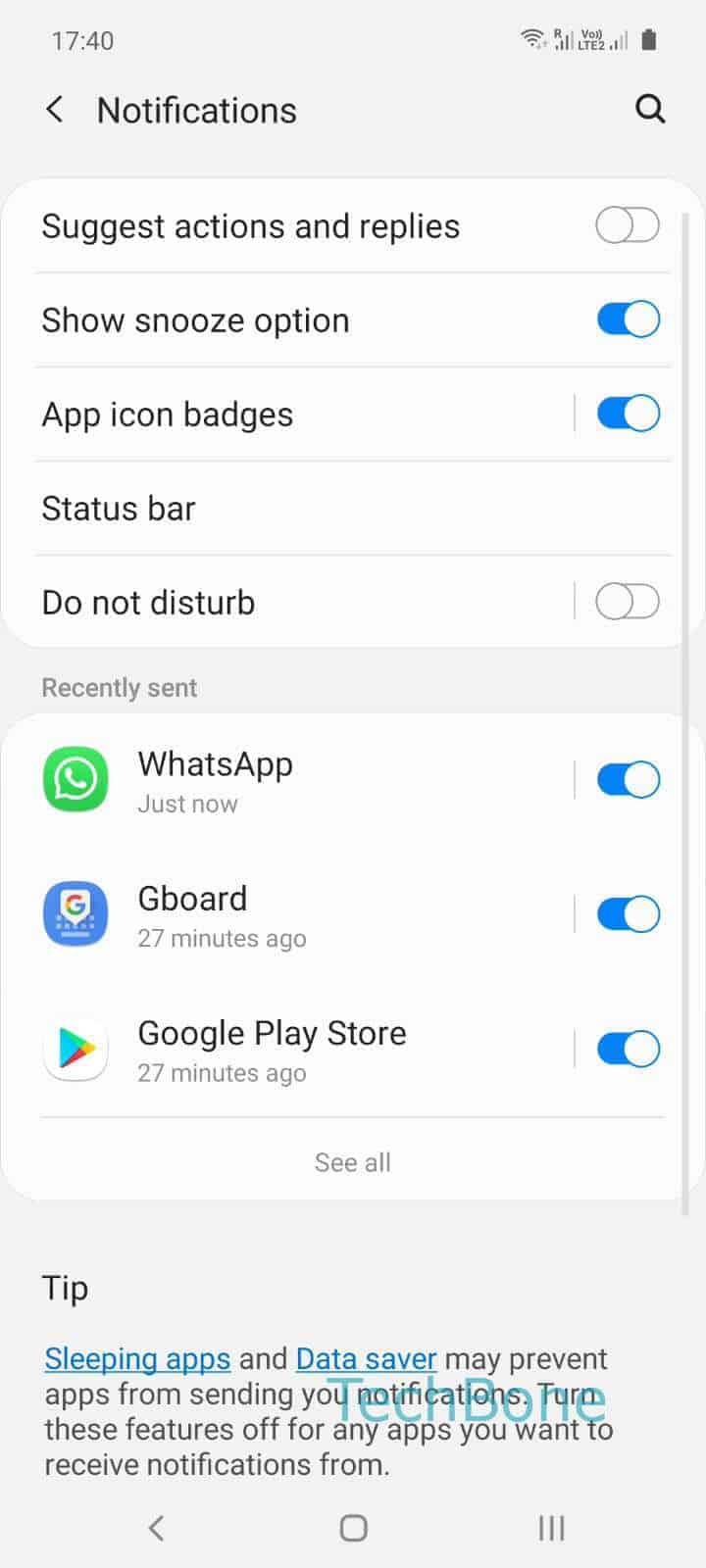Caption:

A cell phone screenshot with a gray background. In the upper left corner, the time is displayed in a darker gray. On the upper right are icons for battery, reception, and Wi-Fi. Two lines down on the left is a black, left-pointing arrow next to the word "Notifications" in black, while a black magnifying glass icon is on the far right. Below this is a white square containing five lines of information, each separated by a light gray line, and four have a toggle switch on the right. The lines read as follows: "Suggest actions and replies" (toggle off), "Show snooze option" (toggle on), "App icon badges" (toggle on), "Status bar" (no toggle), and "Do not disturb" (toggle off). 

Beneath this section is another gray background patch with "Recently sent" written in small gray text. This is followed by another white square containing icons and toggle switches for "WhatsApp," "Gboard," and "Google Play Store," all set to the on position. Centered below this white square in gray text is the option "See All." 

At the very bottom, on the left, the word "Tip" is in black, followed by text explaining that "Sleeping apps" and "Data Saver" (both blue and underlined) may prevent apps from sending notifications. It advises turning these features off for apps you want to receive notifications from.